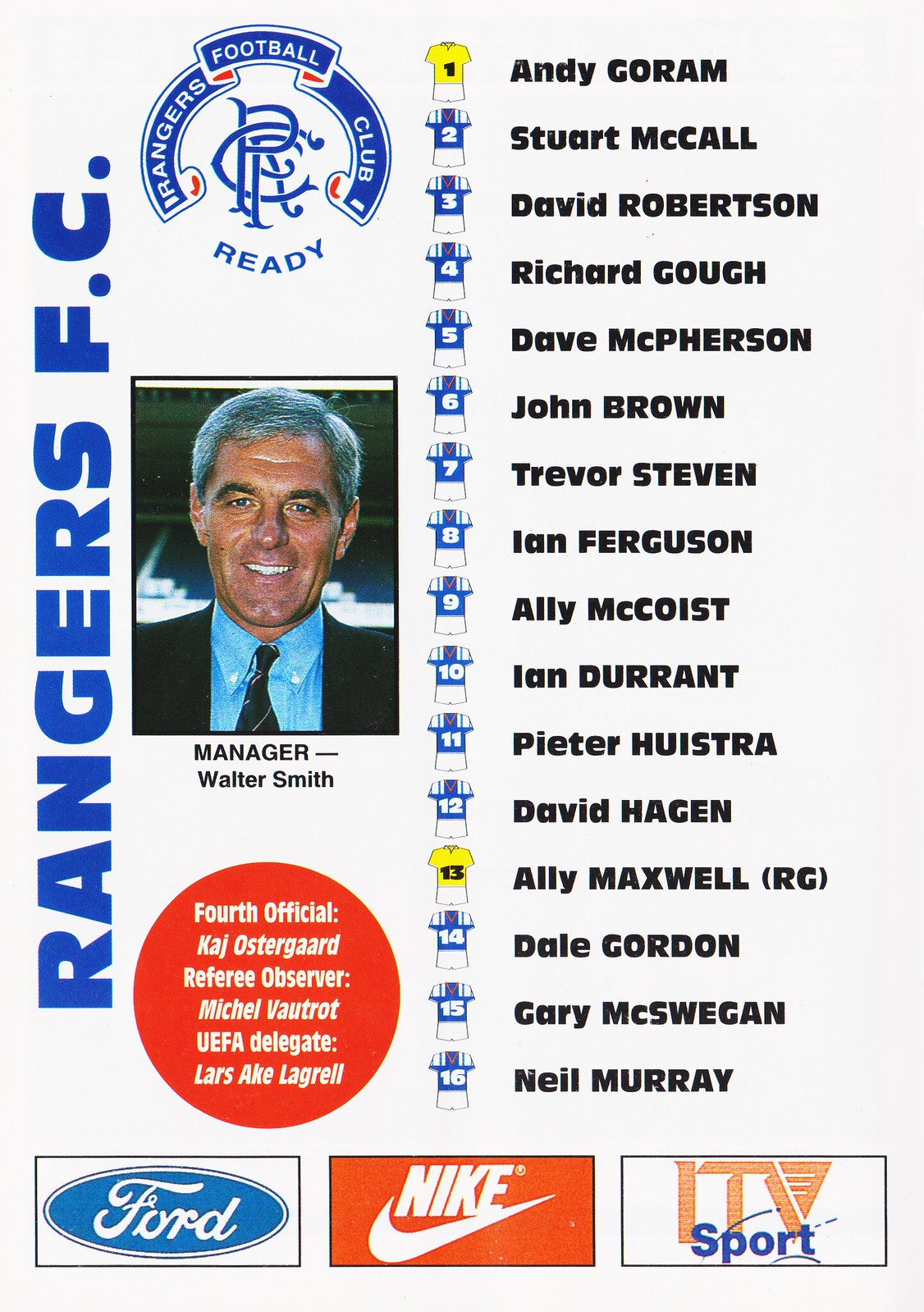The image is a detailed scan of a program page from an old magazine for the soccer club Rangers FC. The left side of the page features the club's name, "Rangers FC," written vertically in a deep blue font. At the top left corner, there is an intricate and stylized club emblem with the letters "RFC" intertwined within a circle, surrounded by the words "Rangers Football Club" and the motto "Ready." Below the logo, there's a centered photograph of Walter Smith, the manager, identifiable by his gray hair and attire of a blue shirt, black jacket, and tie, standing in a football stadium. His name, "Walter Smith," is labeled underneath the photograph.

To the right side of the page, there is a list of players, each associated with jersey numbers. A red circular section below the manager's name highlights official and observer information for the game, including Fourth Official Kaz Ostergaard, Referee Observer Michael Valtrat, and UEFA Delegate Lars Aklagro. 

The bottom section of the page displays the logos of the club's main sponsors: Ford, Nike, and ITV Sport. The combination of photographic realism and graphic design typography lends the program page a polished and professional appearance.